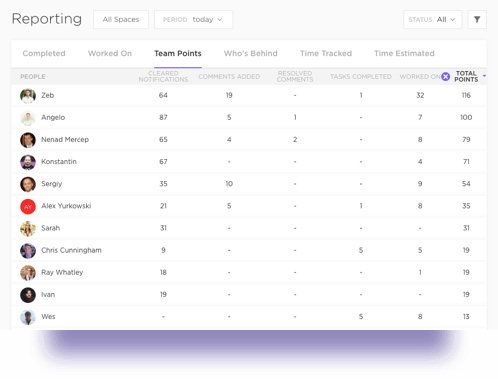This screenshot displays a detailed reporting dashboard. At the top, there's a header labeled "Reporting" with a filter option set to "Today". Below, the interface contains six columns labeled as follows: "Completed," "Worked On," "Team Points," "Who's Behind," "Time Tracked," and "Time Estimated". The main area of the dashboard features a table listing approximately twelve users, each identified by a username and a small profile picture next to it. The users appear to be ranked based on combined metrics from the columns, which include indicators such as comments added, resolved comments, and tasks completed. This layout seems designed to provide a comprehensive overview of team productivity and individual contributions in a clear and organized manner.